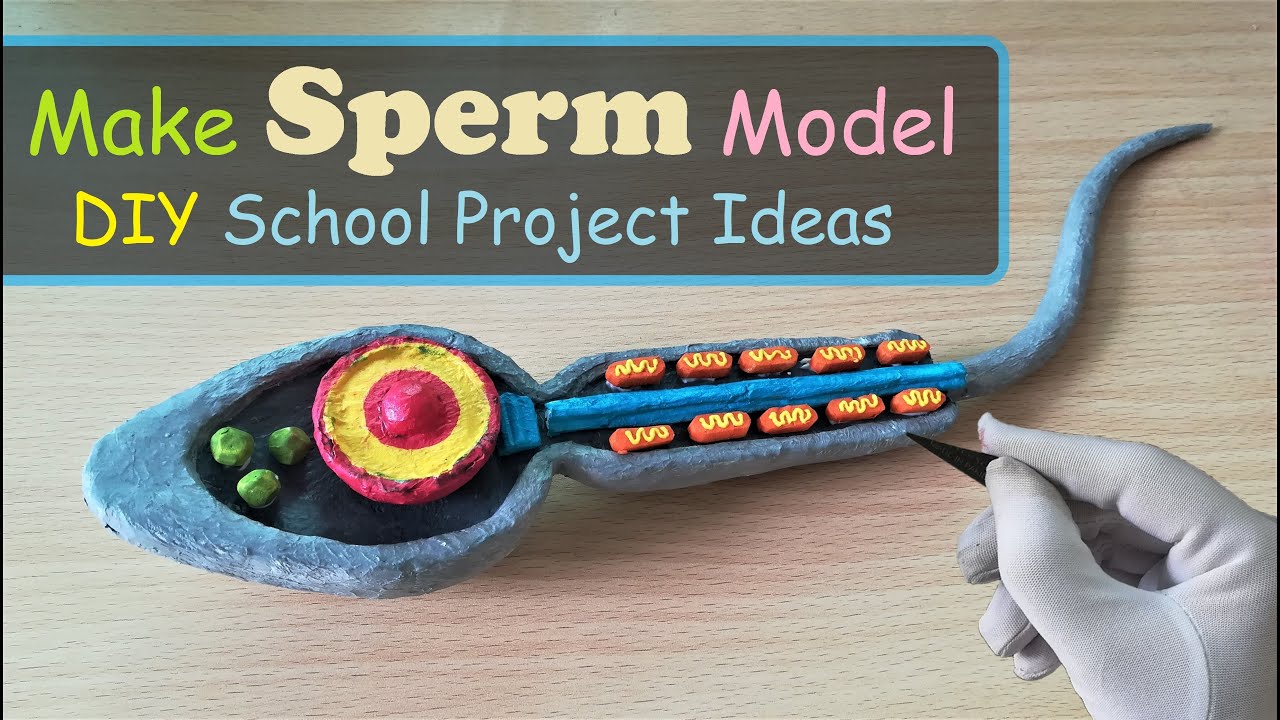This photograph showcases a detailed, handcrafted model of a sperm cell, serving as a do-it-yourself school project idea. It features various colored texts on the left side that read "Make Sperm Model" in green, "DIY" in pink, and "School Project Ideas" in blue. The model itself, crafted from clay, prominently displays a vivid blue exterior stretching from the head to the tail, with a darker blue ridge running along the tail. The head of the sperm contains intricate details, including three small green dots and a distinctive round structure filled with a red center and yellow outer ring, bordered by red. Inside, jagged yellow lines on orange segments add further intricacy. Below the model, which rests on a wooden table surface, a gloved hand in the bottom right corner uses a black scalpel, seemingly refining the details of this educational creation.